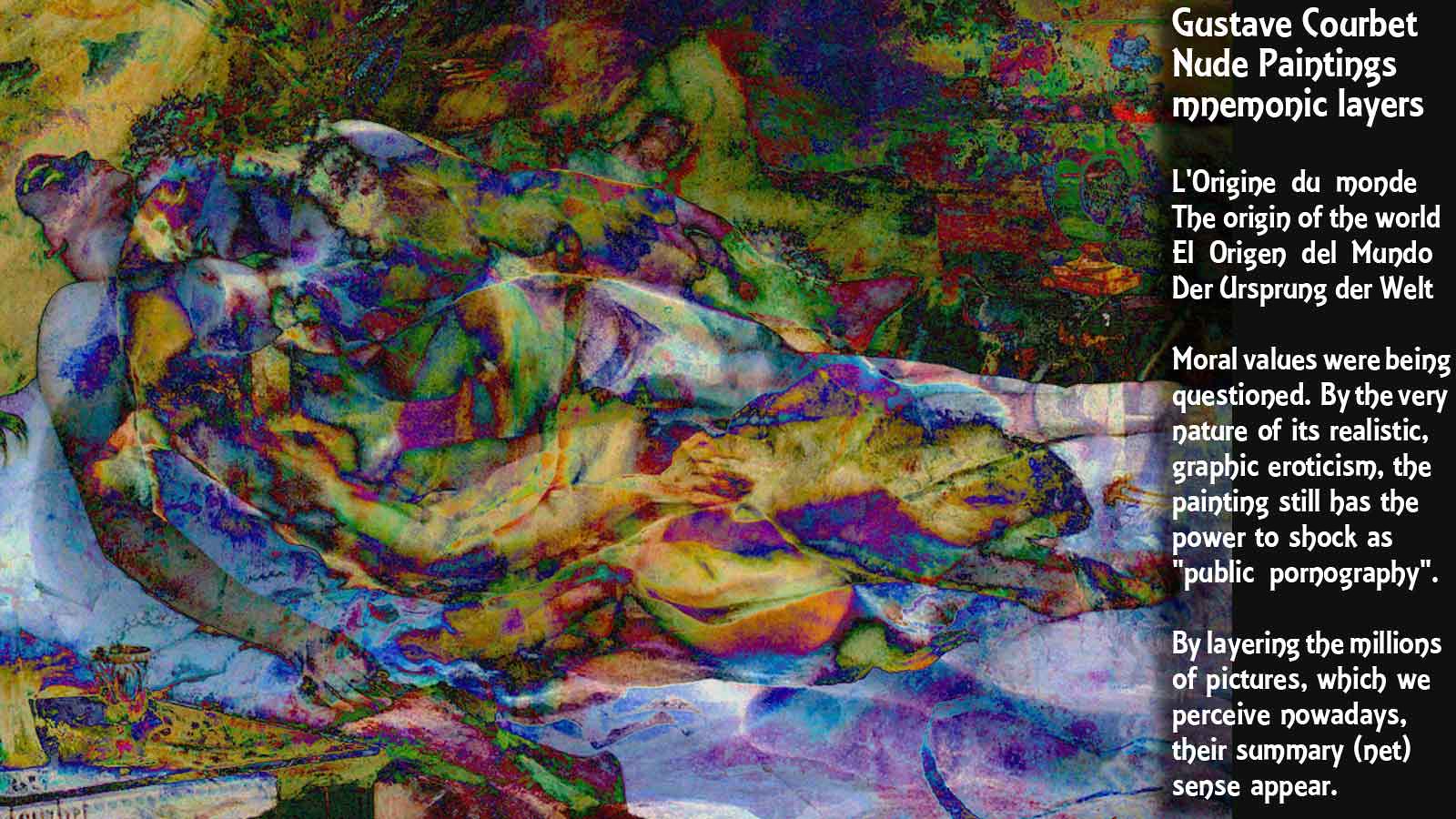The artwork, attributed to Gustave Courbet, is a composite of photography and painted media, predominantly abstract. The painting is positioned horizontally, with the left side consumed by a vibrant, blotchy composition featuring vivid colors such as yellow, green, red, purple, and blue. This overlay of colors forms an indistinct image that seemingly depicts a person, possibly two, lying supine, with an ambiguous object on top of them. 

On the right side of the page, a black rectangular bar contains a description in white text. The text, presented both in English and French, reads: "Gustave Courbet, Nude Paintings, Mnemonic Layers." It mentions that moral values were questioned by the painting's realistic and graphic eroticism, maintaining its shocking impact akin to public pornography. It also notes the modern context of the work, referring to the overwhelming layering of millions of images we perceive today, summarizing in a "net sense." Additionally, various translations of "The Origin of the World" are included. 

The piece, with its blend of abstract forms and vibrant colors, evokes a sense of chaotic yet discernible imagery, challenging perceptions and conjuring a multitude of interpretations through its layered visual and textual presentation.